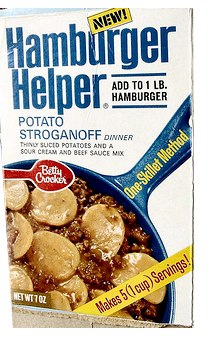This image features an antique box of Hamburger Helper, likely from its original release. The box is predominantly white, with various labels and text adorning its surface. At the very top, a yellow tab with the word "NEW" stands out, indicating it is a newly introduced product at the time. Below this, the product name "Hamburger Helper Potato Stroganoff" is printed in blue lettering.

Prominently displayed on the box's front is an illustration of a black cast-iron skillet, containing a mixture of ground beef and scalloped potatoes, demonstrating the meal that can be prepared using the contents. The text adjacent to the skillet image highlights the convenience of the "One Skillet Method" and notes that the meal yields "Five 1-Cup Servings." A signature red spoon, featuring the iconic lettering "Betty Crocker" in white, further authenticates the product's branding. The overall design and imagery suggest a nostalgic and retro feel, evoking memories of classic home-cooked meals.